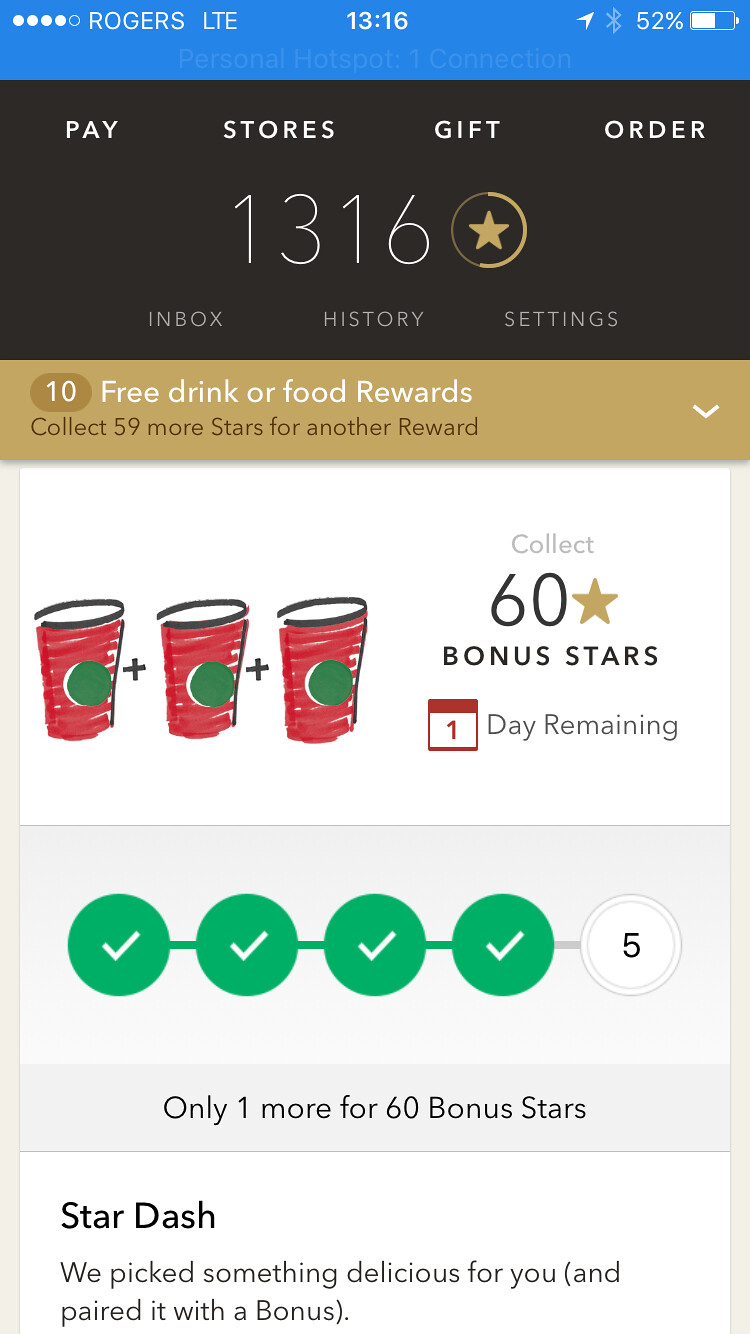The image depicts a color screenshot from a food app on a phone screen. At the top, there is a blue banner displaying five circles, four of which are white, along with text in all caps saying "Rogers LTE." On the right side of the blue banner, there is an arrow symbol and a 52% battery indicator. Below the banner, in a black rectangle with white capital letters, are the options: "PAY STORES GIFT ORDER." The time is indicated as 13:16 (1:16 PM) in the middle of the screen.

Further down, there is a section displaying the user's current point balance of 1316 with a star icon. Below this are smaller navigation options: "Inbox," "History," and "Settings." A brown banner follows, showing "10" with the text "Free drink or food rewards." Underneath, it's mentioned in black print that collecting 59 more stars will earn another reward.

There is an illustration of three cups with plus signs between them, indicating a "Collect 60 bonus stars" offer with "one day remaining" noted below. Further down, there are four green circles with white check marks inside, and an additional fifth empty circle. The text says "Only one more for 60 bonus stars." At the bottom, there is a mention of "Star Dash" with the note: "We pick something delicious for you and pair it with a bonus."